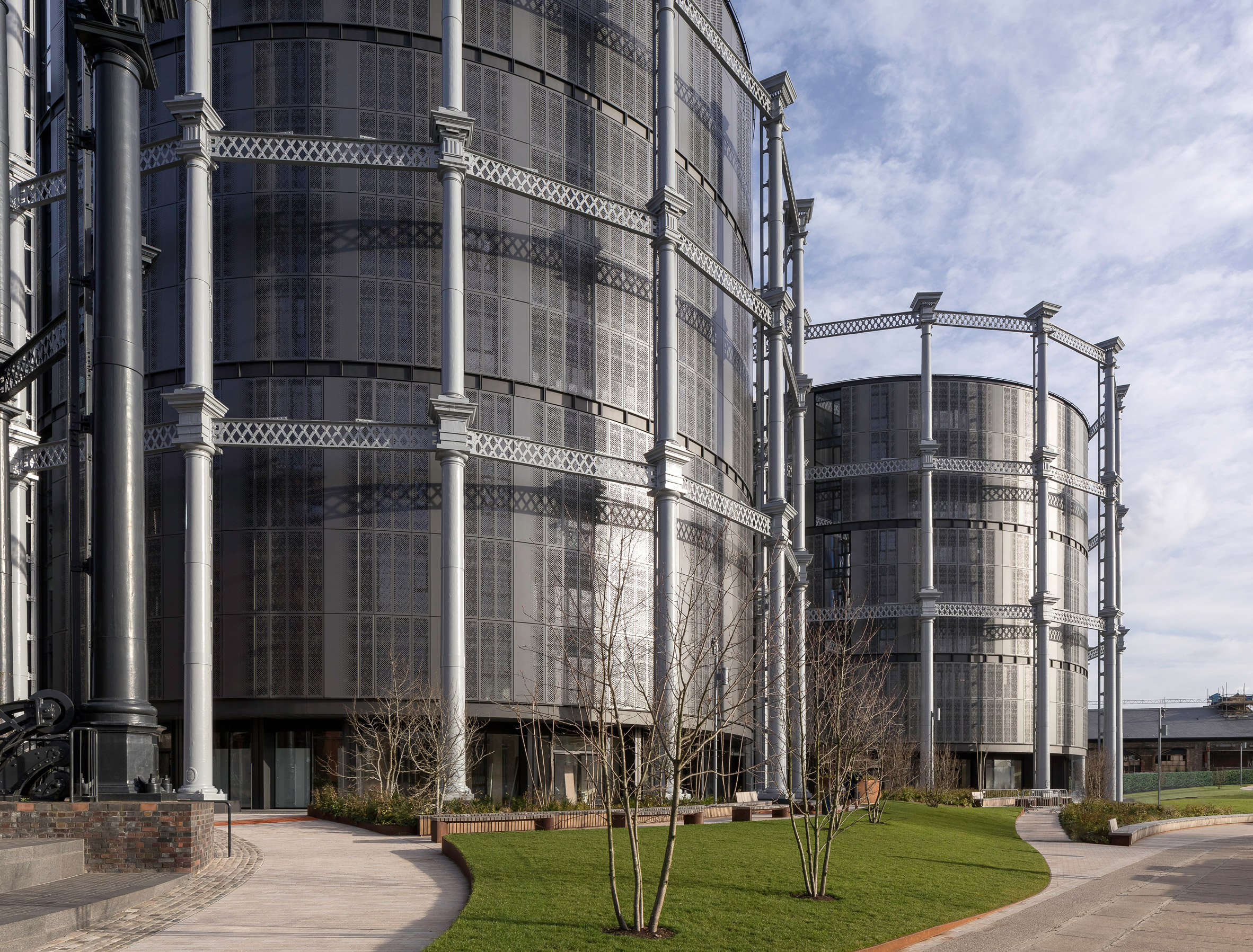The image depicts an expansive outdoor area dominated by tall, silver-colored buildings with a distinctly industrial design. These structures are adorned with conspicuous steel columns that form a grid-like pattern across their exteriors, imparting an appearance of reinforced metal framework. Among the buildings, the most prominent ones are cylindrical in shape, with metal frameworks and visible ladders running along their sides, suggesting an industrial or scientific facility, perhaps even a brewery. 

In the foreground, a neatly paved gray sidewalk winds through patches of vibrant green grass, while along the walkway, there are benches for sitting. The landscape also includes a few orderly planted trees and small grassy areas that intersperse the built environment. Additionally, the image captures a section of the roadway on the lower right and a small, rectangular building positioned to the far right. The sky overhead is a light blue, with white clouds scattered throughout, adding to the scene's overall openness and expansive feel.